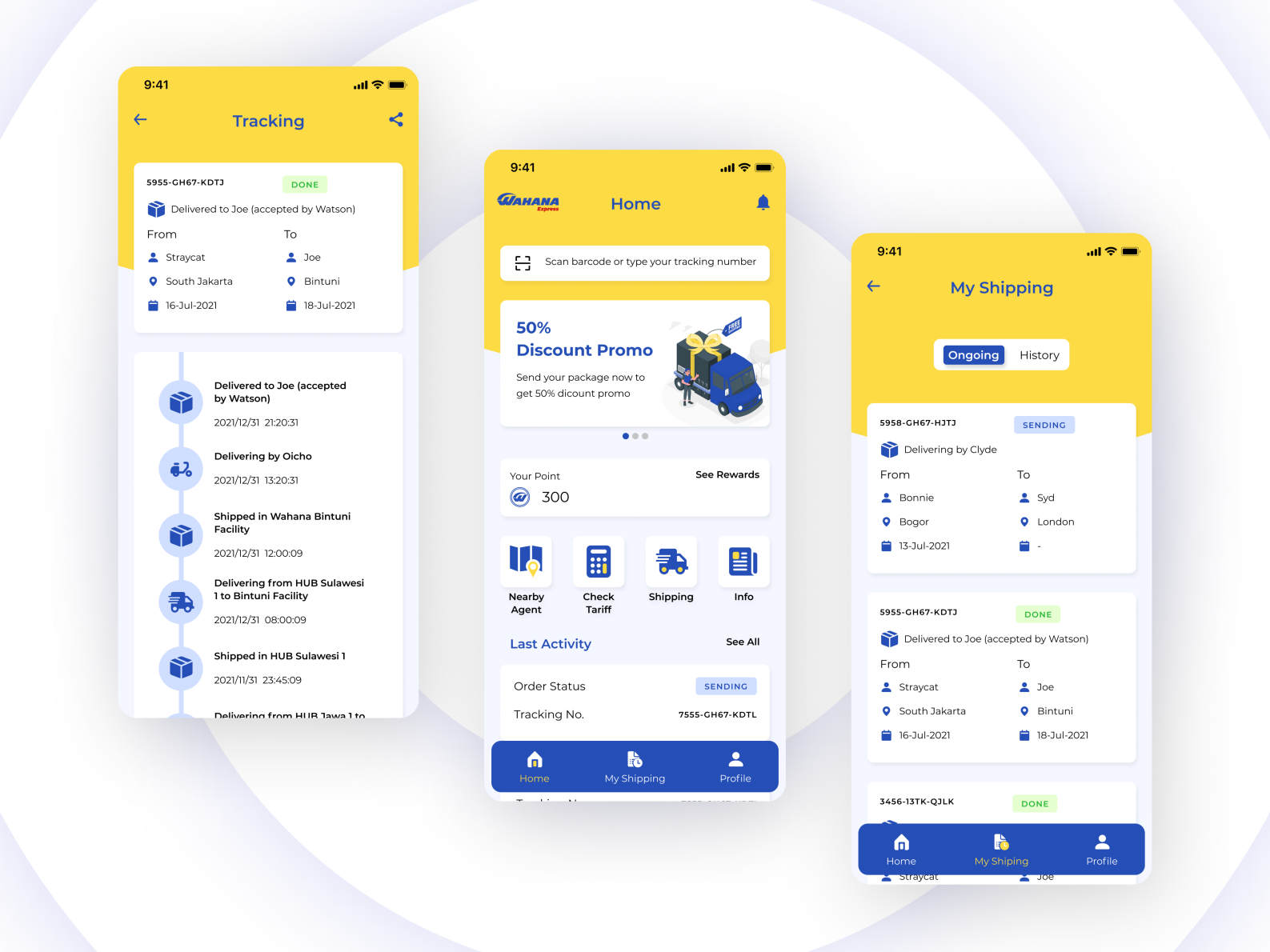The image displays a smartphone screen segmented into three sections. The top portion is divided into two areas: the top-right and top-left, while the center and bottom-right sections form the rest of the layout. The background features two distinct colors—yellow at the top and light blue at the bottom, with a central dividing section in green.

At the top of the image, the text reads: "Trekking delivered to Joe, accepted by Watson from Stray Cats, location South Jakarta. Day 16, July 2021." Further down, it indicates: "To Joe, location Bintuni, Date 18, July 2021." A progress bar is visible, showing the delivery's current status as delivered to Joe, accepted by Watson, delivered by Oiko, and shipped via Wahana from Hub Sulawesi to Bintuni.

The second page details the interface of the Wahana Express app. It features a QR code scanner or an option to type a trekking number. A promotional message offers a 50% discount, written in blue text. Another text prompts users to send their packages to avail of the discount. User points are indicated as 300. Several blue buttons with different functions are displayed, including "Nearby Agent," "Check Tariff," and "Shipping Info." At the bottom, there are status updates such as "Last Activity" and "Order Status: Sending," along with a trekking number. The bottom navigation includes buttons for "Home," "My Shipping Profile," with a blue background, indicating their height. On the left side, options for "My Shipping Ongoing" and "History" are visible.

The final section addresses another shipment: "Shipment sending, delivered by Clyde from Boni, location Bongo, Date stated, July 2021, to Seat, location London. The delivery date is still pending. A completed shipment is marked as 'done,' showing it was delivered to Joe by Watson, identical to the completed shipment details on the left side."